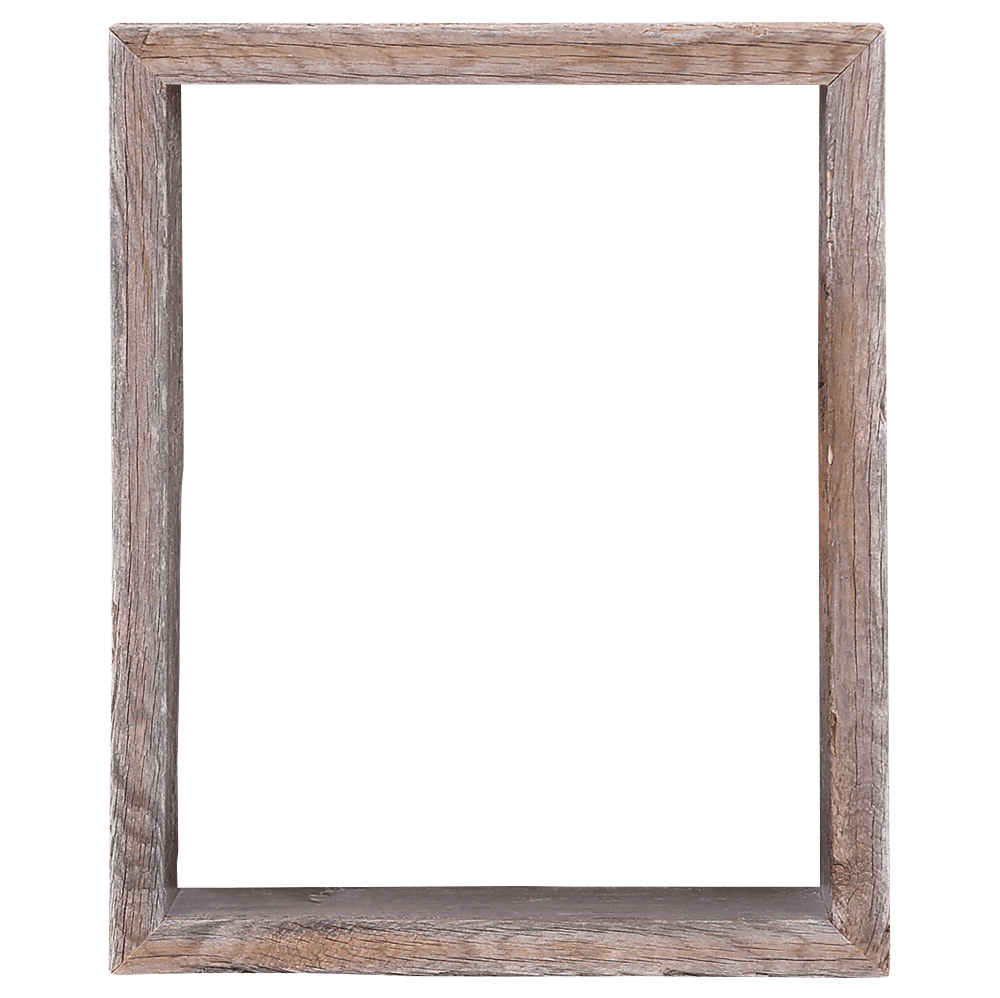This image showcases a rustic, rectangular picture frame set against a pure white background, giving the illusion it is floating in an empty space. The frame is crafted to mimic rough-hewn, untreated wood, presenting a dried, weathered appearance with visible cracks along the edges. The natural wood texture of the frame displays variations in color from light gray to brown, contributing to its aged and rustic aesthetic. Each of the four sides of the frame exhibits unique color characteristics: the top bar, being the lightest, features subtle white spots, while the left and right sides are similar yet distinct, with the right side showing a slight brown tint in the center and the left side leaning towards a darker brown hue. The bottom piece blends both brown and dark brown tones but presents more dark brown shades compared to the right side. Both the inner and outer edges of the frame reveal these intricate wood colors and details, further enhancing its vintage, handcrafted look. Inside the frame remains a vertical white rectangle, mirroring the same empty white void as the background, emphasizing the frame's solitary presence in the image without any surrounding distractions or inserted image.